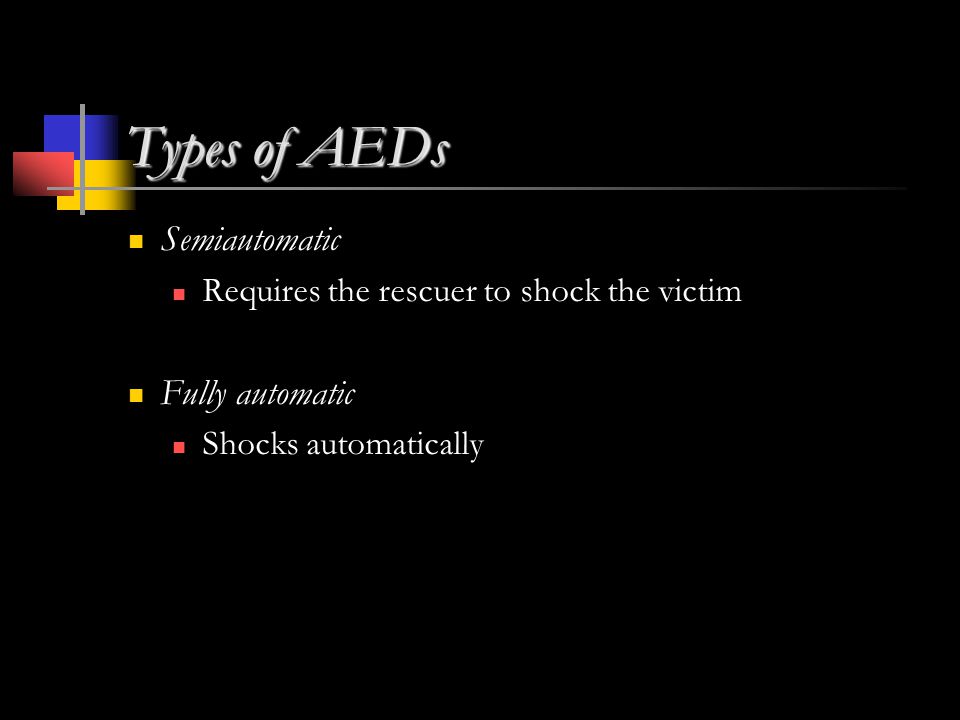This large, square image features a solid black background and resembles a digital presentation slide, likely designed in PowerPoint. In the upper left corner, there's a combination of a title and a logo. The logo itself consists of three layered rectangles; the top one is blue, the left one is red, and the right one is yellow. Adjacent to this logo, the title "Types of AEDs" is displayed in gray font. A short vertical gray line sits to the left of the title, with a long horizontal gray line extending from beneath it, fading off to the right. Below this header, the slide features two main bullet points marked with yellow squares. The first yellow bullet point reads "Semi-automatic," with an indented red sub-bullet point stating "Requires the rescuer to shock the victim." The second yellow bullet point reads "Fully automatic," accompanied by a red sub-bullet point that says "Shocks automatically." The colors used in the slide include black, white, gray, blue, red, and yellow, contributing to its clean and professional appearance. The textual content is strategically placed in the upper and middle portions of the slide, providing clear information about the types of AEDs.